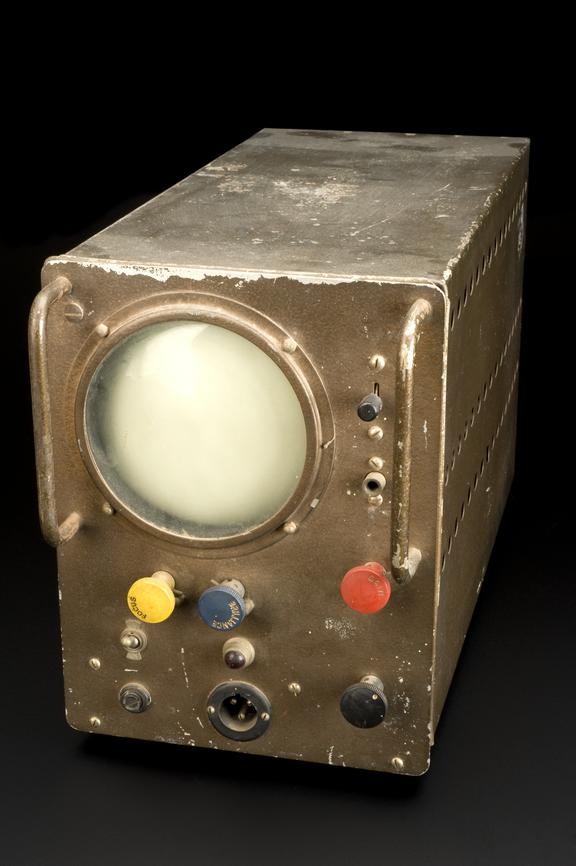This photograph shows an aged, rectangular box-like device with a black background, possibly set against a black table or backdrop. The device, resembling an oscilloscope, is gold or brown in color but has significant paint wear, appearing white and dusty on the top and scratched on the front. Two metal handles are attached to the left and right sides, providing grip. On the right side are three rows of holes, likely for air ventilation. The front of the device features several buttons: a yellow button on the left, a blue button in the center, a red button on the right, positioned higher than the others, and a black button below. At the top, there's a circular, creamy white screen or lens, suggesting it might be a viewing or output component. The device is the size of a toaster and shows extensive signs of use and damage, indicating it is quite old.